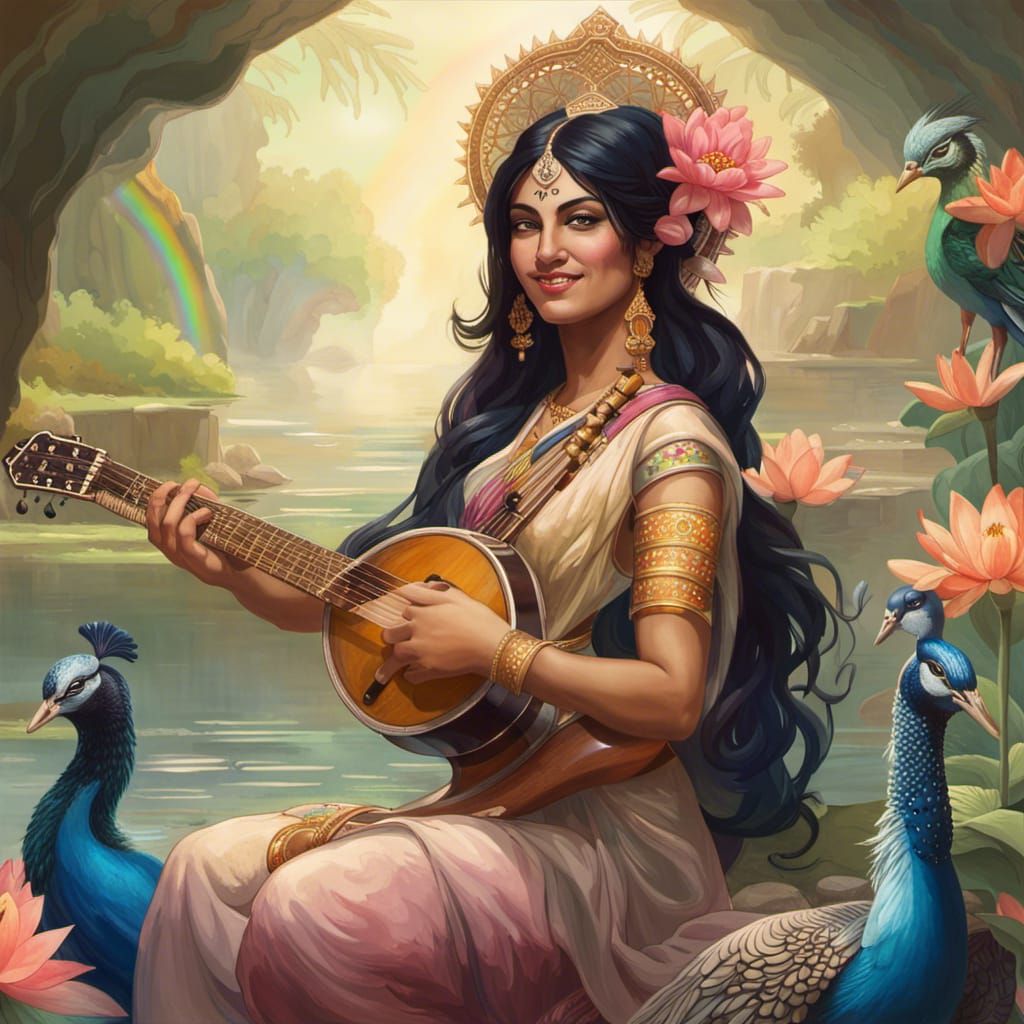This highly stylized, possibly AI-generated, anime or digital illustration depicts a serene, captivating scene centered around a woman dressed in traditional Indian attire. She wears a light pink and gold sari, adorned with bracelets, a golden armlet, and a delicate headpiece with flowers in her long, flowing dark hair. She is seated in the foreground, smiling and engaged with a stringed instrument, resembling a mandolin or banjo, with her left hand mid-strum.

Flanking her are two majestic blue peacocks, while a smaller bird perches higher up on her shoulder. The setting appears to be a tranquil cave beside a stream or lagoon, with pale-colored water and waterfalls forming a serene backdrop. Above her, an arched stoneway frames the scene, leading the viewer’s eye to the lush trees, vibrant flowers, and a softly glowing rainbow on her left-hand side. The combination of these elements evokes a sense of calm and ethereal beauty.